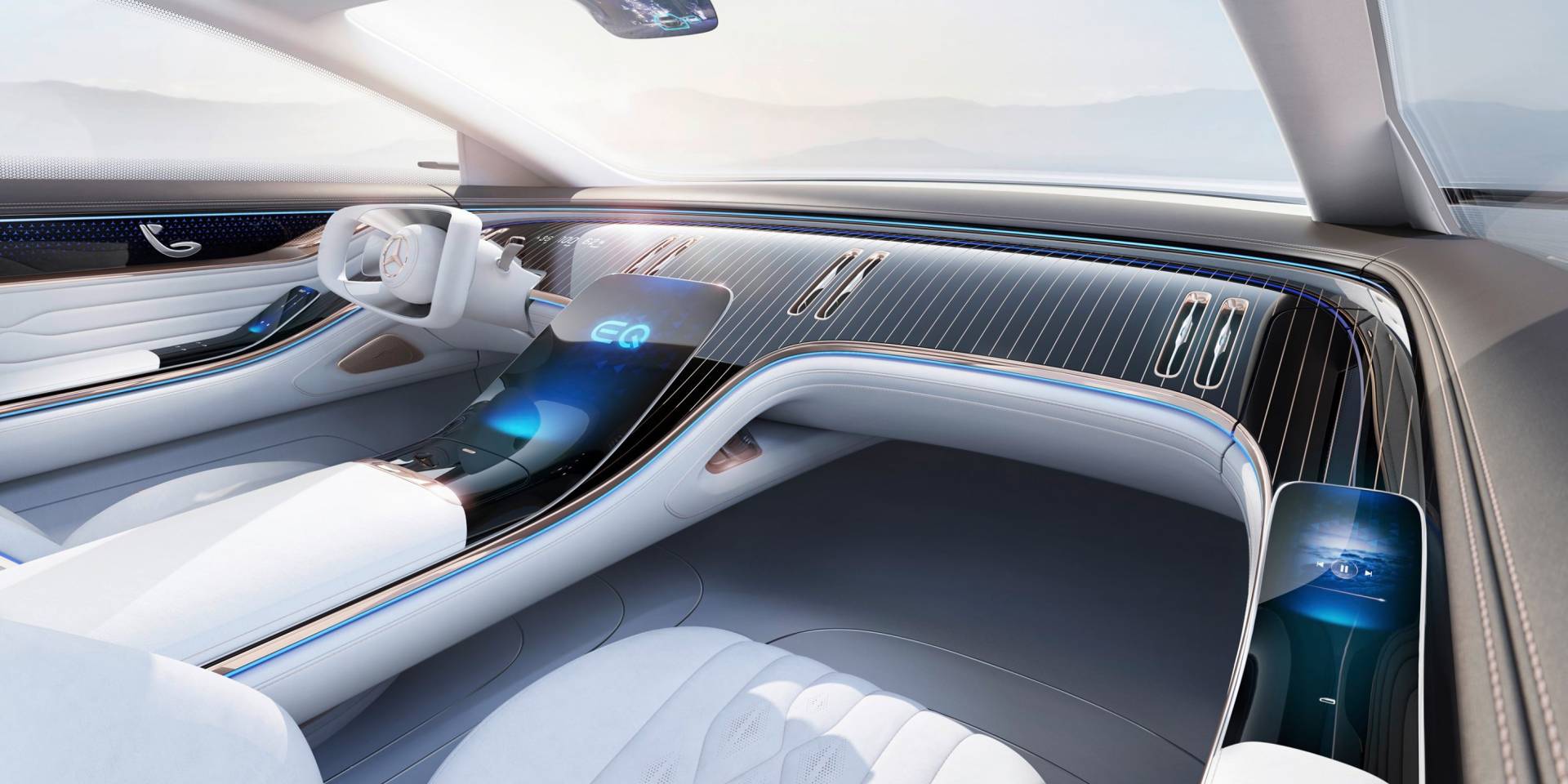This image showcases the ultra-modern interior of a futuristic Mercedes-Benz EQ coupe. The design strikes a balance between luxury and forward-thinking technology. The front and passenger seats are crafted from sleek white leather, emphasizing a pristine, almost sterile aesthetic, complemented by a glossy, black dashboard adorned with vertical lines that resemble a pinstripe suit. Notably, these stripes have been described as both thin white lines and vertical gold lines, contributing to the interior's dynamic visual appeal.

The centerpiece of the dashboard features a cutting-edge digital console in a sleek light blue and black finish, while additional screens are integrated into the doors, offering both the driver and passenger seamless access to controls. The driver’s experience is highlighted by a distinctive square steering wheel bearing the iconic Mercedes logo at its center. This rectangular wheel, matching the car's futuristic theme, is situated on the left-hand side, with the adjacent control panel accommodating various seat and mirror adjustments.

In front of the seats, a broad windshield reveals a faint mountain range bathed in bright light, enhancing the sense of openness and cutting-edge exploration. The absence of visible air vents adds to the streamlined, clean design ethos. This interior, poised for the future, epitomizes the sleek, luxurious direction of Mercedes-Benz's forthcoming electronic coupe.